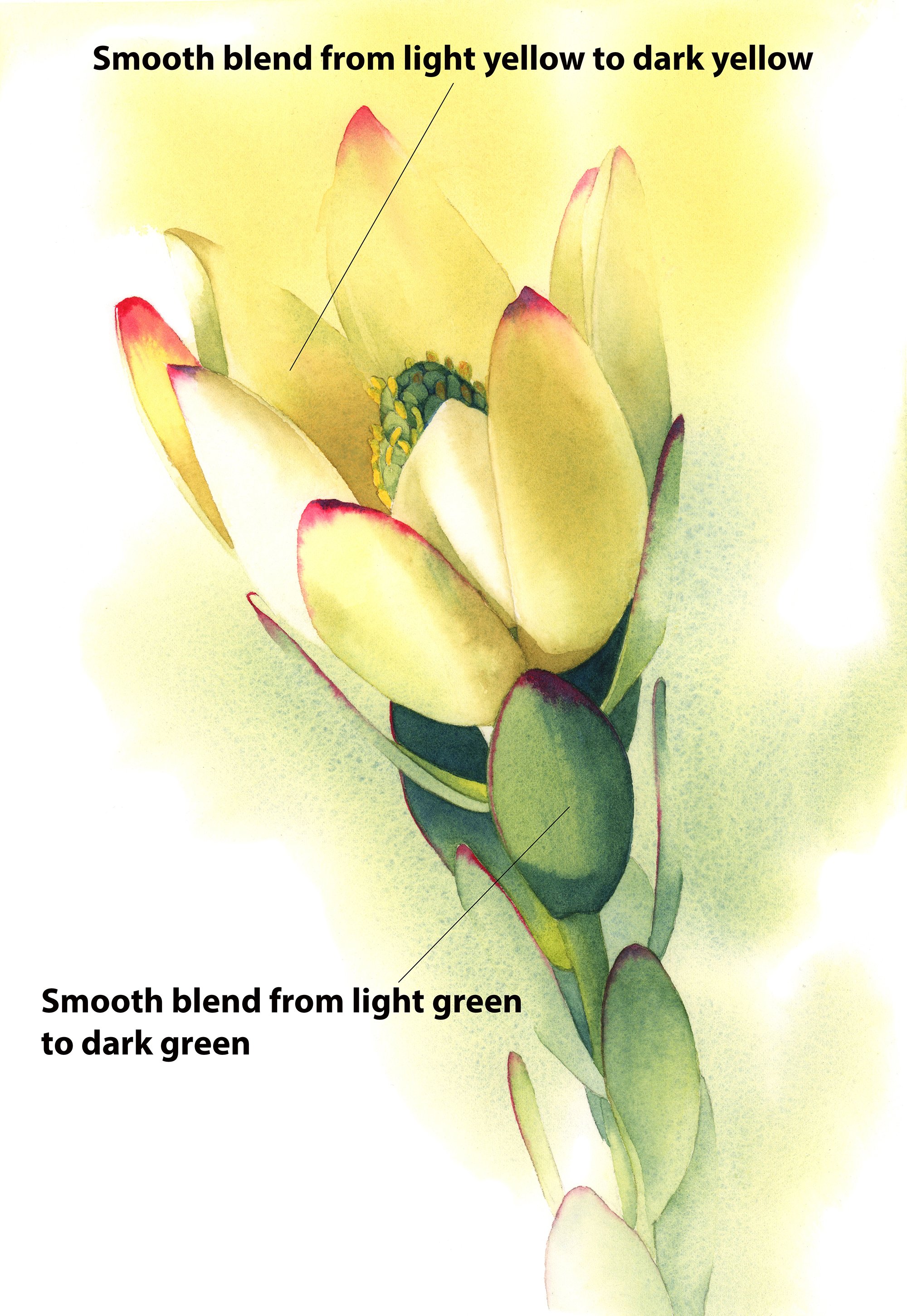This illustration, possibly done with colored pencils or in a watercolor-like style, depicts an open flower with detailed shading instructions. The flower features rounded, yellow petals with reddish tips and a greenish-yellow aura surrounding them. At the top, black text reads, "smooth blend from light yellow to dark yellow," indicating a gradient transition in the petal's coloring. The flower's core is bluish-green. Green leaves with a slight red tinge on the tips extend from the stem, and similar in shape to the petals. At the bottom, text points to the leaves and states, "smooth blend from light green to dark green," illustrating a color gradient in the leaves. The image serves as a labeled diagram or guide for shading colors in a drawing or painting.